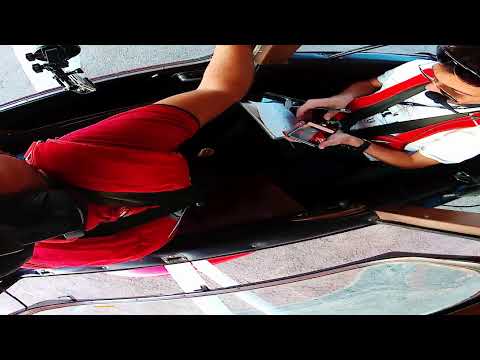A distorted photograph taken from an odd angle captures two individuals in what appears to be a bus, with black borders at the top and bottom of the image. One person, standing towards the back, wears a red shirt with black lining on the sleeves, black pants, black suspenders, and has a backpack with red straps; they appear to be looking at a notebook held in their right hand while holding a pencil in their left. They also have what seems to be a black camera strap. The second individual, partially obscured, stands closer to the bus door, wearing a white shirt with black and red suspenders, and appears to be facing left. They also sport sunglasses, which might be doubled due to the distortion. The bus door handle is visible at the bottom right of the image, reinforcing the sense that both individuals are waiting to exit the bus. The photo's curvy distortion gives an impression of cramped space, with both people appearing somewhat squished together.